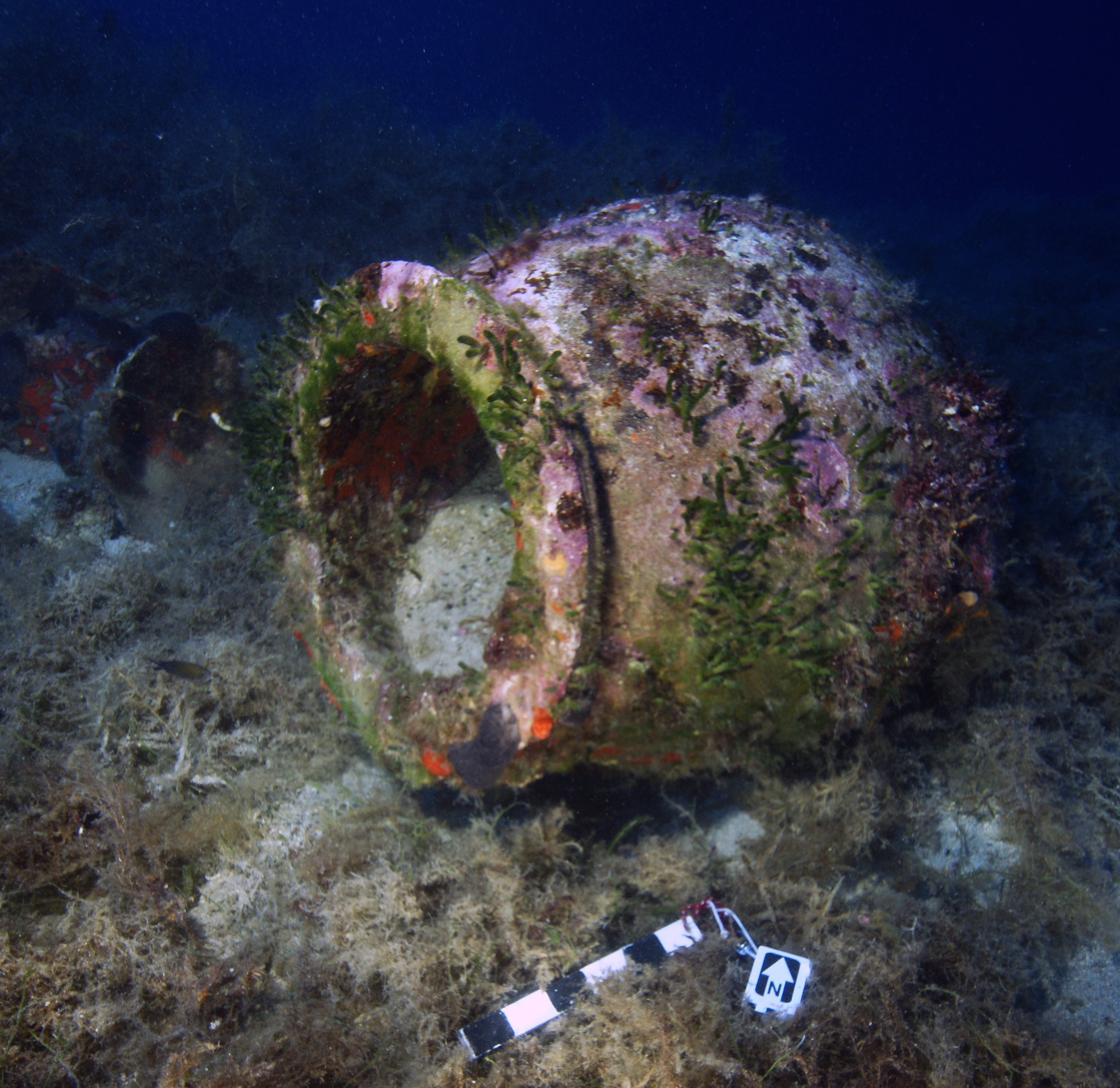The photograph depicts an underwater scene dominated by a large, ancient urn or vase, crafted from what appears to be brown terracotta. The vase lies on its side with its opening facing left, partially buried in the sandy ocean floor. The subdued colors of the vase are mostly brown, accented by patches of purple and red corrosion or marine growth. The vase is richly adorned with green algae, moss, and various underwater plants, signaling a lengthy submersion in its watery grave. The background water is a dark indigo, lending an air of deep-sea mystery to the entire setting. Near the base of the vase, a black and white striped marker, reminiscent of a movie director’s clapboard, is laid out. Attached to it with a small metallic carabiner is an identification tag bearing a north-pointing arrow and the letter 'N', presumably for cataloging purposes. This setup reinforces the notion that the artifact is part of an organized archaeological investigation.